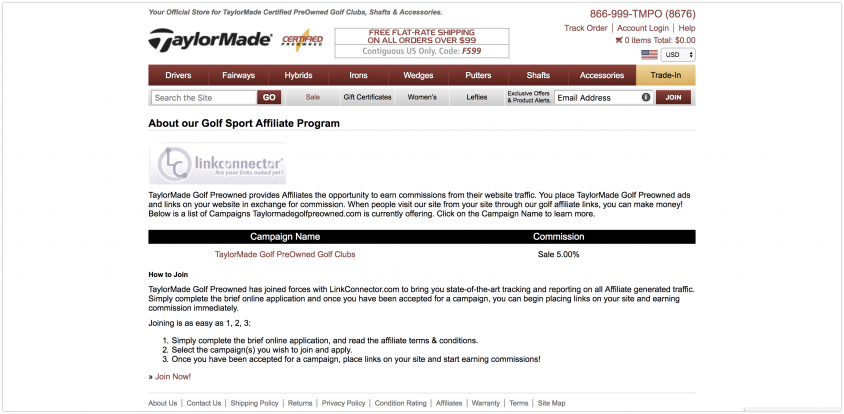**Descriptive Caption:**

This screenshot captures the homepage of a website specializing in TaylorMade certified pre-owned golf clubs, shafts, and accessories. The background is predominantly white, providing a clean and uncluttered appearance. Across the top of the page, there is a prominent banner stating, "Your Official Store for TaylorMade Certified Pre-Owned Golf Clubs, Shafts, and Accessories." Below this message, the site's logo is displayed in large black font: "TaylorMade." The "T" in "Taylor" is rendered in white and set within a black guitar pick-shaped area. Adjacent to the logo is a certification emblem with a yellow slash through it indicating authenticity.

Further down, a promotional banner announces, "Free Flat Rate Shipping on All Orders Over $99 - Contiguous US Only," followed by the discount code "F599." To the right of this banner, there is a customer service phone number: "866-999-TMPO (8676)."

Directly beneath the promotional and contact information, the site offers quick access links: "Track Order," "Account Login," "Help," and a shopping cart status showing "0 Items - Total $0.00." An American flag icon denotes the currency as USD, with a dropdown menu for changing the payment method, although the site only ships within the contiguous US.

A brown navigation bar spans the width of the site, functioning like a site map, with categories including: "Drivers," "Fairways," "Hybrids," "Irons," "Wedges," "Putters," "Shafts," and "Accessories." There is also an option for "Trade-In."